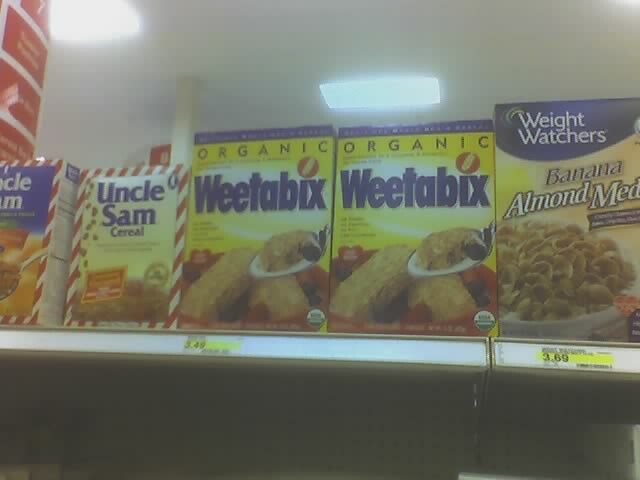In this brightly lit grocery store aisle under fluorescent lights, the top shelf displays a variety of cereals. Dominating the shelf are boxes of Weight Watchers Banana Almond Medley, priced at $3.69, and two boxes of organic Weetabix at $3.49 each. The Weight Watchers boxes feature a blue, white, and tan color scheme, while the Weetabix boxes showcase a mix of blue, yellow, red, and tan, matching the cereal's color. An Uncle Sam cereal box is also visible among them, and there’s an additional cereal box at the very edge, partially obscured, making it difficult to identify its brand or type. Each price is clearly marked on yellow and white stickers positioned beneath the corresponding cereal boxes.